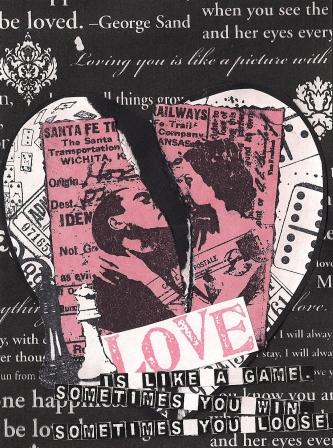This is a color photograph of an artistic collage set against a black background. Dominating the center is a torn white heart, overlaid by a pink illustration of a man and woman kissing. Both the heart and the kissing couple are torn apart, with the man and woman split down the middle. Surrounding this central focus are multiple quotes written in white, including the prominent phrase, "Love is like a game. Sometimes you win. Sometimes you lose." The word "love" is prominently displayed in pink with a white banner. The collage also features words like "Santa Fe" and "always," and the fragmented background includes elements resembling dominoes and letters cut out from magazines. The meticulous placement and tearing of these elements suggest a deeply emotive, almost scrapbook-like piece of art that conveys the fragile and unpredictable nature of love.